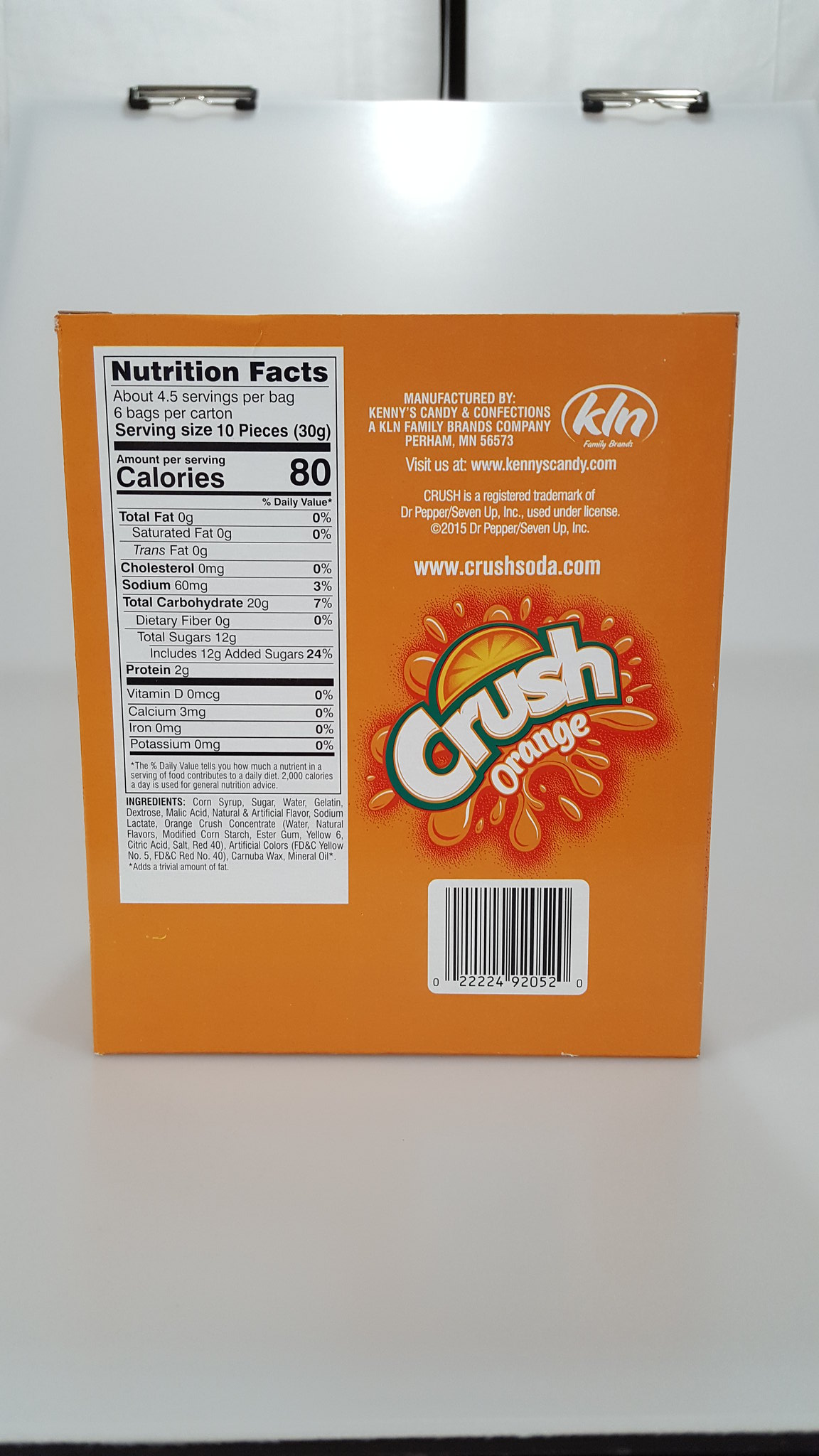The image displays the back of an orange Crush package, prominently featuring the Crush logo in white text, outlined in black with a sun-like motif and orange squiggles surrounding it. The background is a light gray surface, likely a table or clipboard, with a light bulb shining from above. The nutritional facts label is positioned on the left-hand side, providing detailed information: each package contains 80 calories, zero total fat and cholesterol, 60 milligrams of sodium, 20 grams of carbohydrates, 12 grams of sugars, 2 grams of protein, and 3 milligrams of calcium. The package includes a QR code at the bottom for scanning. Additional text indicates it's manufactured by Kenny's Canadian Confections, part of the Kale and Family Brands Company, based in Perham, Minnesota. The image also faintly shows some cloth or wall in the background with a black pole, yet the focus remains on the detailed description of the Crush Orange packaging.